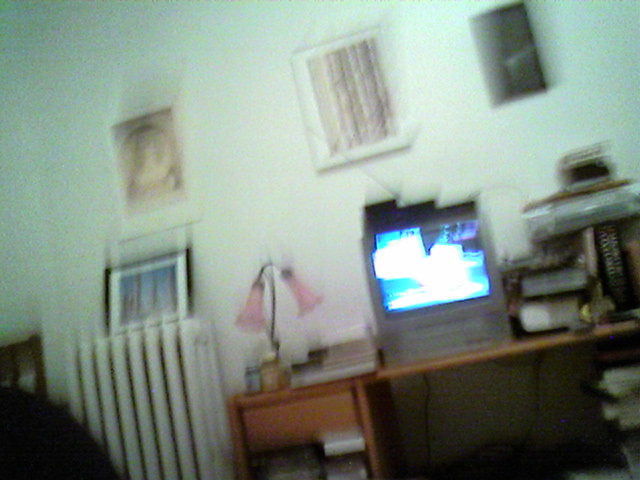This photograph, taken from within a home, captures a cozy, albeit slightly blurry and distorted, corner of a room. The centerpiece of the scene is a wooden desk resting against a white wall. Dominating the desk is an older, square-shaped television set with a built-in VCR at its base, its gray exterior contrasted by the indistinct blue lights on its screen. To the right of the TV, several books are neatly stacked. On the left side of the TV sits a charming lamp adorned with pink, flower-like accents, casting a gentle light. Further to the left, additional books are piled, and a wooden drawer is visible beneath them. Scattered around the desk are a few vitamin bottles, adding a touch of daily life to the setting. The backdrop features a plain white wall, adorned with a picture frame, a vent, and various small accessories, completing this intimate snapshot of a lived-in space.